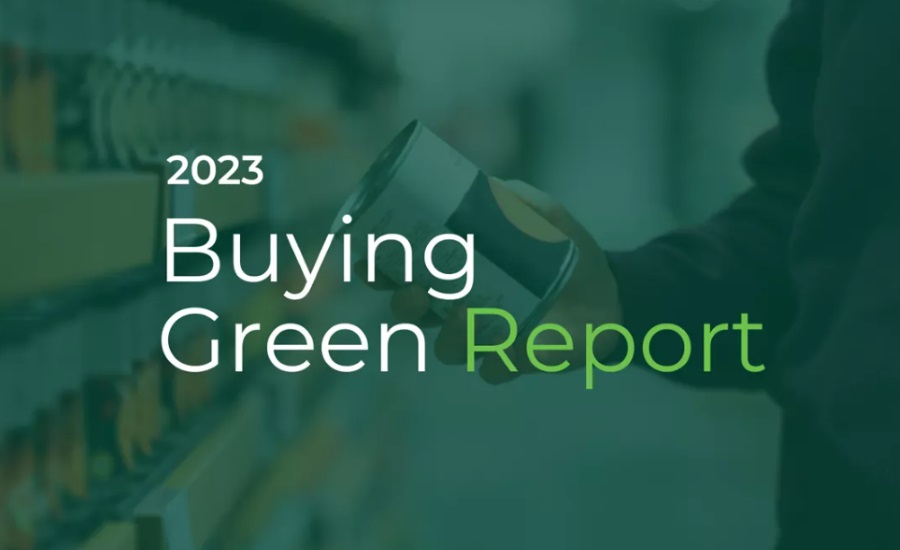The image is a landscape-oriented color photograph, prominently featuring the text "2023 Buying Green Report" in white, with "report" highlighted in a lime green color. The entire image is cast in a translucent hunter green tint. A woman, partially visible on the right, stands in a grocery store, holding a can of food in her right hand. The can is white-labeled, with a black box at the bottom and an orange circle within the box. The woman's dark-colored shirt appears influenced by the green hue, making the exact color indeterminate. Behind her, the store shelves are stocked with various indiscernible products. An indistinct person is visible in the blurred background. The artistic style blends photographic realism with special effects filters and superimposed text, conveying a modern, eco-friendly theme.